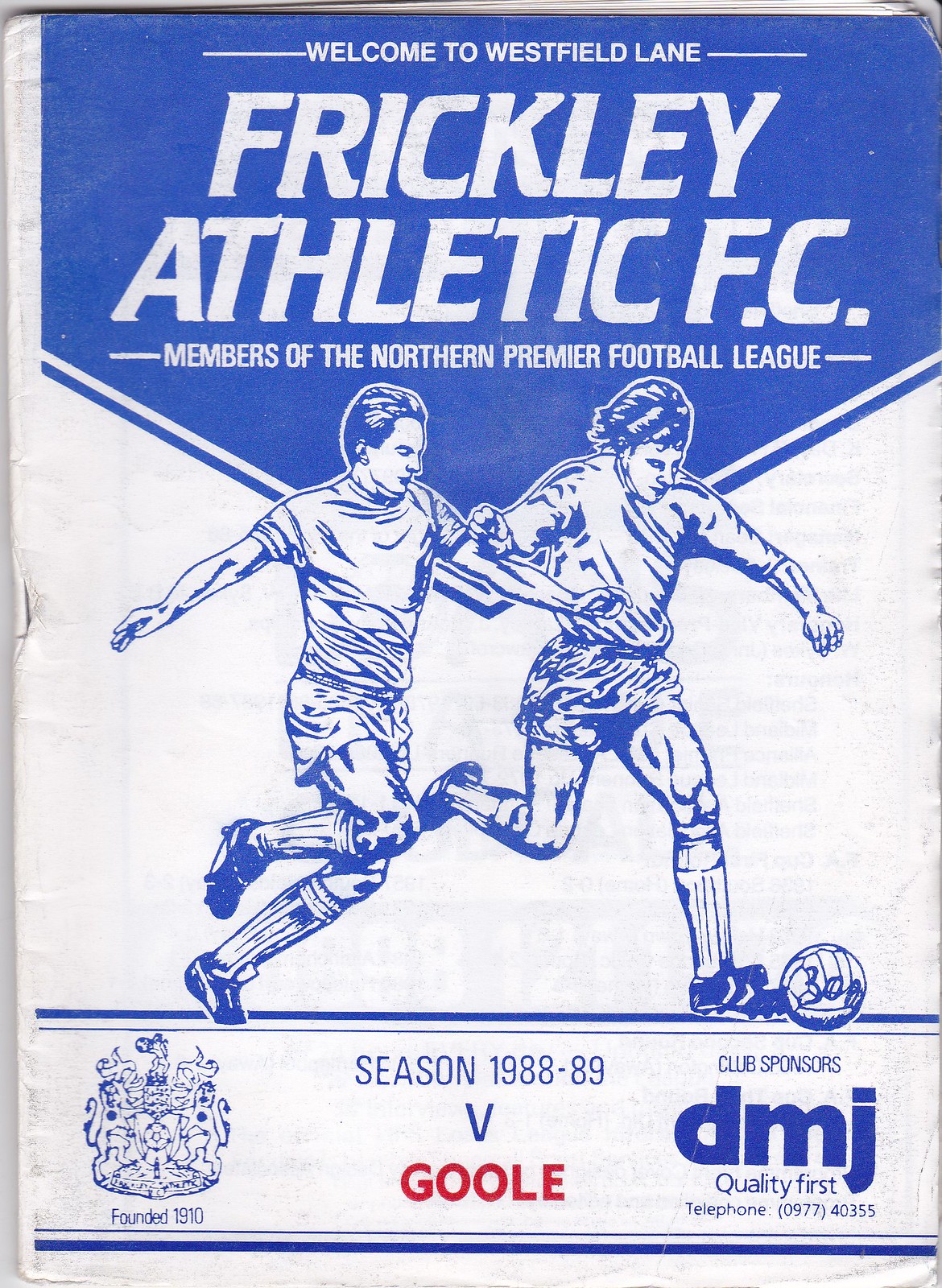The image is designed as an advertisement for a soccer game, featuring predominant blue and white colors. At the top, a blue badge tapers towards the middle, displaying in white text: "Welcome to Westfield Lane," followed by "Frickley Athletic FC" in larger capital letters. Underneath, it reads: "Members of the Northern Premier Football League."

Central to the image is a cartoon drawing of two football players from opposing teams, with the player on the right poised to kick the ball. Below the illustration, blue text announces "Season 1988-1989," followed by "versus Goole" in striking red letters.

The top left corner features the football club's logo along with the text "Founded in 1910." In the bottom right, the sponsors are mentioned in blue text: "Club Sponsors DMJ Quality First, Telephone 0977 40355." This detailed depiction emphasizes the match advertisement and all associated elements.